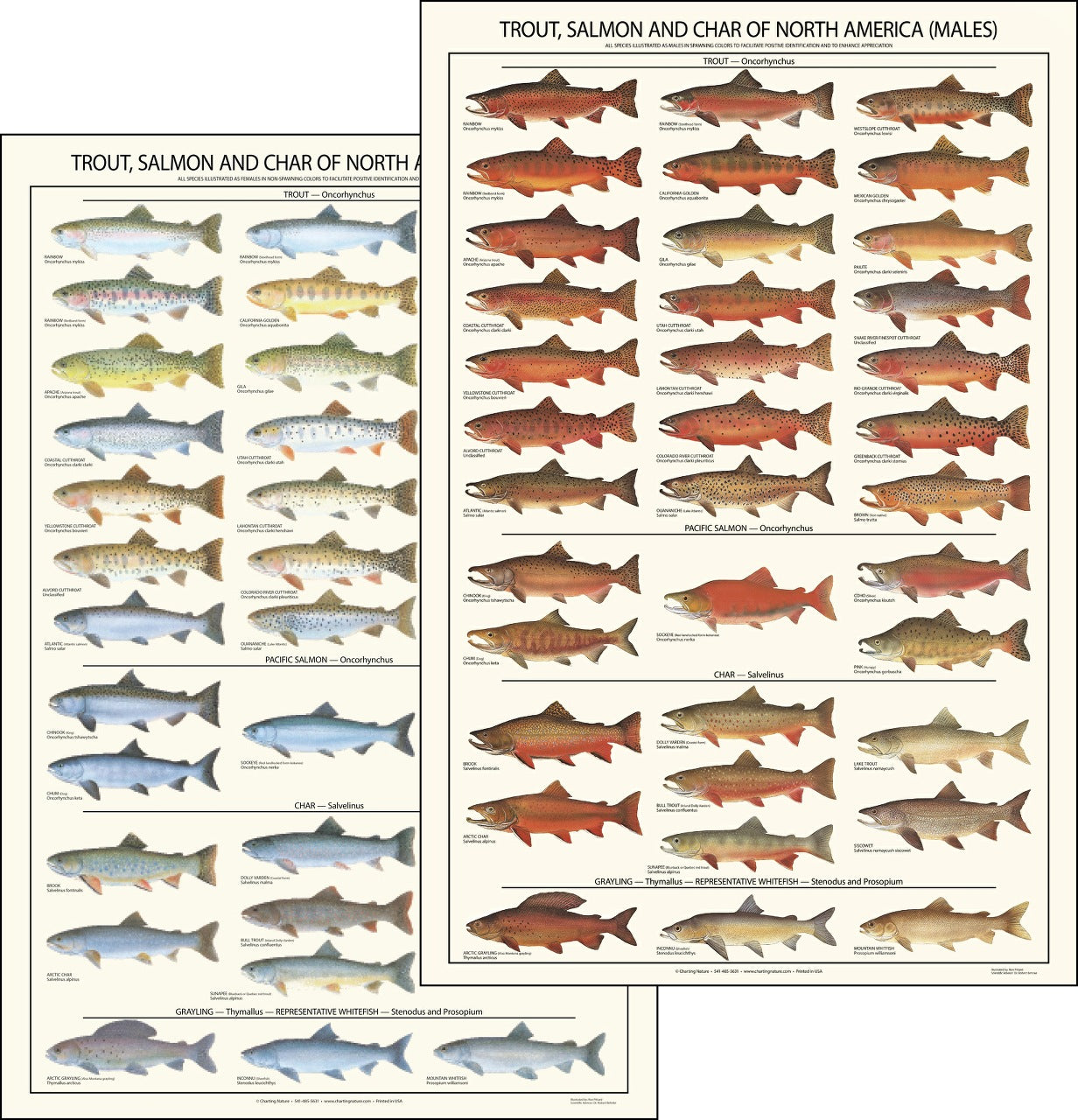This scientific illustration features two vertically oriented, rectangular charts with beige backgrounds, showcasing different types of fish commonly found in North America. The right-hand chart, positioned slightly higher than the one on the left, is titled "Trout, Salmon, and Char of North America (Males)." It displays approximately 20 to 30 images of salmon, trout, and char, organized into three columns. The fish depicted on this chart are predominantly red and brownish, with some possessing orange accents. In contrast, the bottom right corner reveals fish that are whitish and brownish.

The left-hand chart, although partially obscured by the right-hand one, also bears the title "Trout, Salmon, and Char of North America." Unlike their counterparts on the right, the fish on this chart exhibit a broader spectrum of colors, including blues, silvers, light greens, and light reds. These fish appear slightly larger and their vivid color differences suggest a focus on variant coloring, possibly the female species, although the label is partially cut off and unclear. Both charts highlight the diversity and distinctive colorations of these North American fish species, providing a detailed visual comparison.